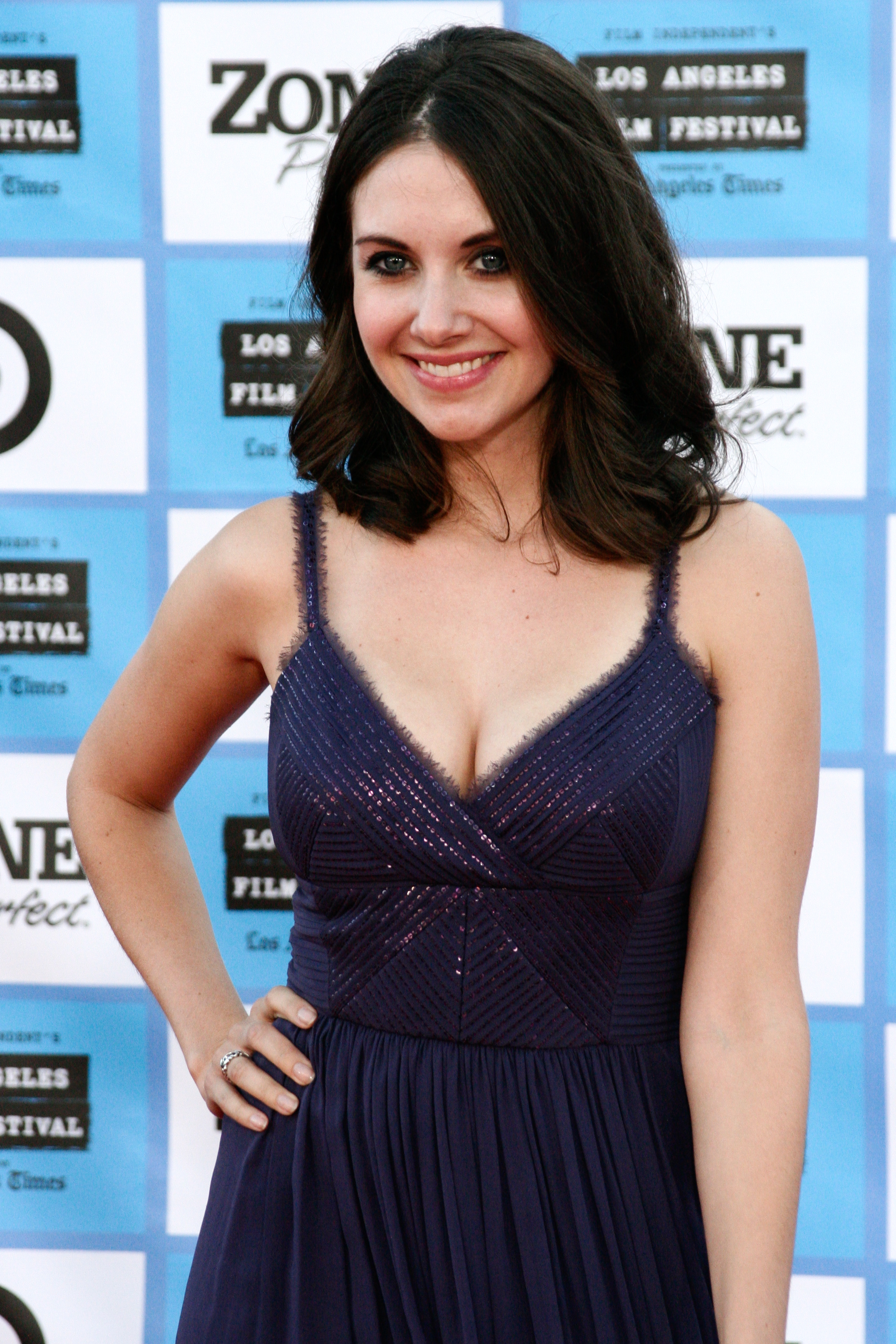In this photograph, Alison Bry is posing confidently at what appears to be a red carpet event. She is capturing attention in a dark navy blue, sparkly, sleeveless dress with a sweetheart neckline. The sparkles are particularly noticeable along the cleavage line and on the strap that ascends the dress, while the bottom half is more frilly and flowy. Alison has her right hand stylishly placed on her hip as she smiles warmly. Her shoulder-length dark brown hair rests casually on her shoulders, and she complements her blue eyes with noticeable dark eye shadow. The backdrop is adorned with blue and white squares featuring various logos, prominently including the Los Angeles Film Festival. She is looking slightly to the left, enhancing her poised and elegant demeanor for the camera.